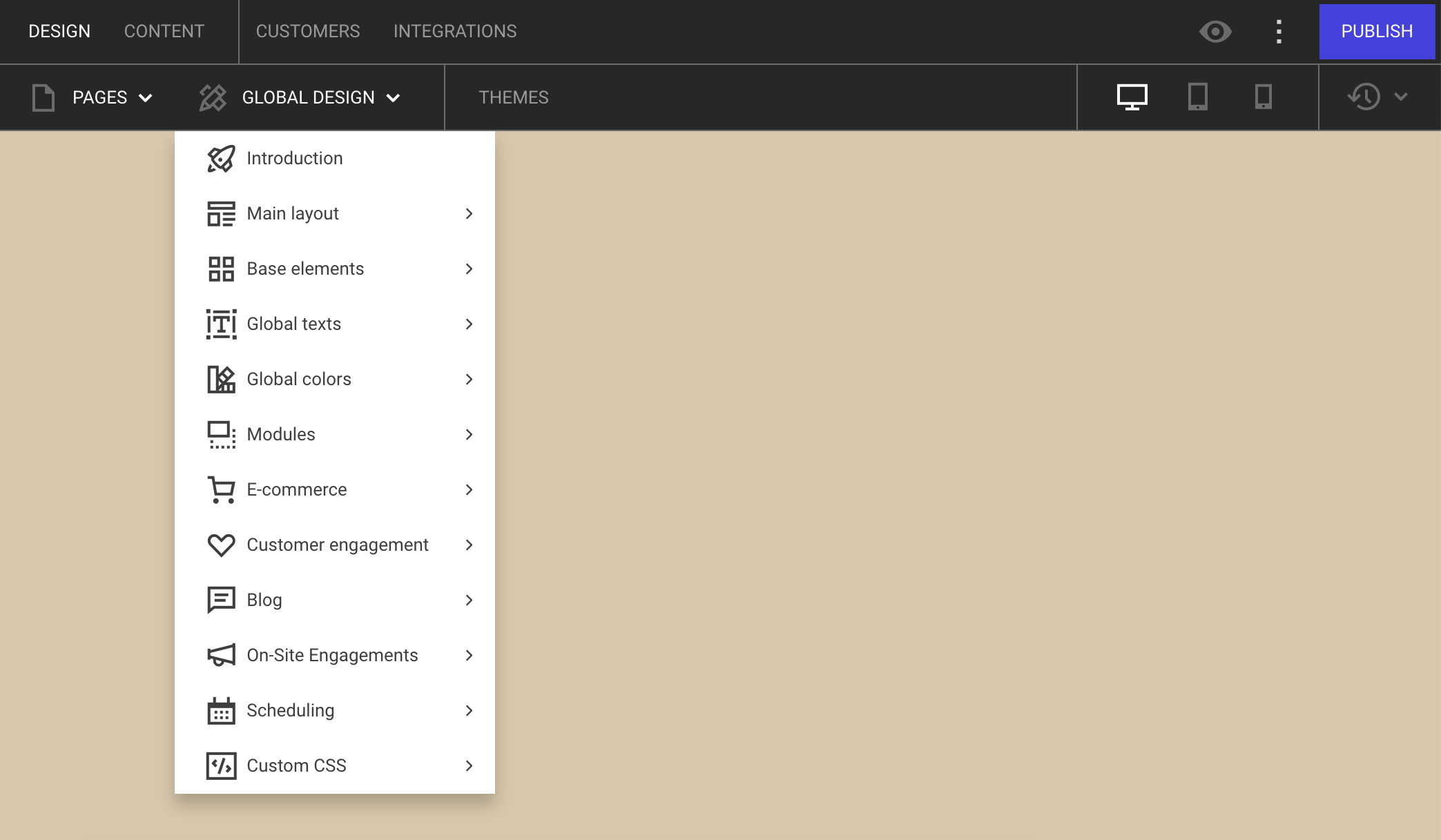The image depicts a user interface of a web design or content management platform. The rectangular page features a black header bar at the top. Positioned on the top left corner of the header, the word "DESIGN" is prominently displayed in white capital letters, followed by "Content," "Customers," and "Integrations," all in regular white font. On the top right corner, there's a blue rectangular button labeled "Publish" in white text.

Below the header, there is an option labeled "Pages" accompanied by a pull-down arrow, and next to it, another option called "Global Design" with a downward-pointing arrow.

The left-hand side of the page contains a vertical column of icons and associated text, representing various sections:
1. A spaceship or small rocket icon labeled "Introduction."
2. An icon resembling a newspaper layout labeled "Main Layout."
3. Four square icons labeled "Base Elements."
4. A "T" icon labeled "Global Text."
5. An L-shaped icon labeled "Global Colors."
6. Two rectangle icons labeled "Modules."
7. A shopping cart icon labeled "E-Commerce."
8. A heart icon labeled "Customer Engagement."
9. A rectangle with text icon labeled "Blog."
10. A bullhorn icon labeled "On-Site Engagements."
11. A calendar icon labeled "Scheduling."
12. A box with arrows pointing left and right labeled "Custom CSS."